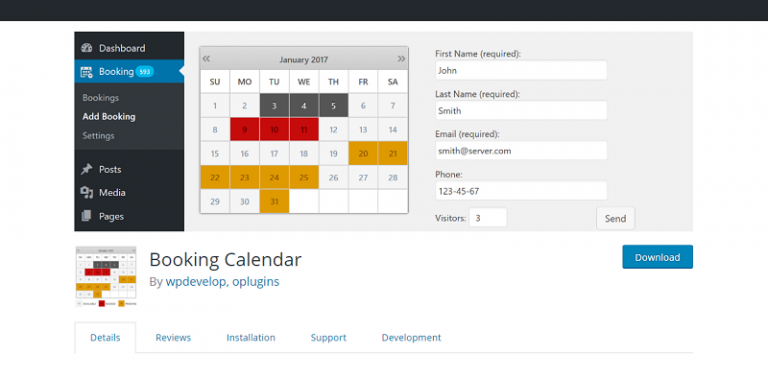A screenshot of a booking calendar website, featuring a black sidebar on the left with white text options including "Dashboard," "Booking," "Posts," "Media," and "Pages." The "Booking" option is highlighted in blue with white text, indicating it's the current selection. To the right, a calendar is displayed for January 2017. Specific dates are color-coded: the 3rd, 4th, and 5th are in black; the 9th, 10th, and 11th are in red boxes; and the 20th, 21st, 22nd, 23rd, 24th, 25th, and 31st are in a dark mustard yellow. 

Adjacent to the calendar is an information box containing fields for "First Name" (John), "Last Name" (Smith), "Email" (smith@server.com), and "Phone" (123-45-67). The "Visitors" count is 3. A "Send" button is present to the right. Below this section is the text "Booking Calendar by WPDevelop.0plugins," accompanied by a blue "Download" button on the right. At the bottom, there are several tabs labeled "Details," "Reviews," "Installation," "Support," and "Development."